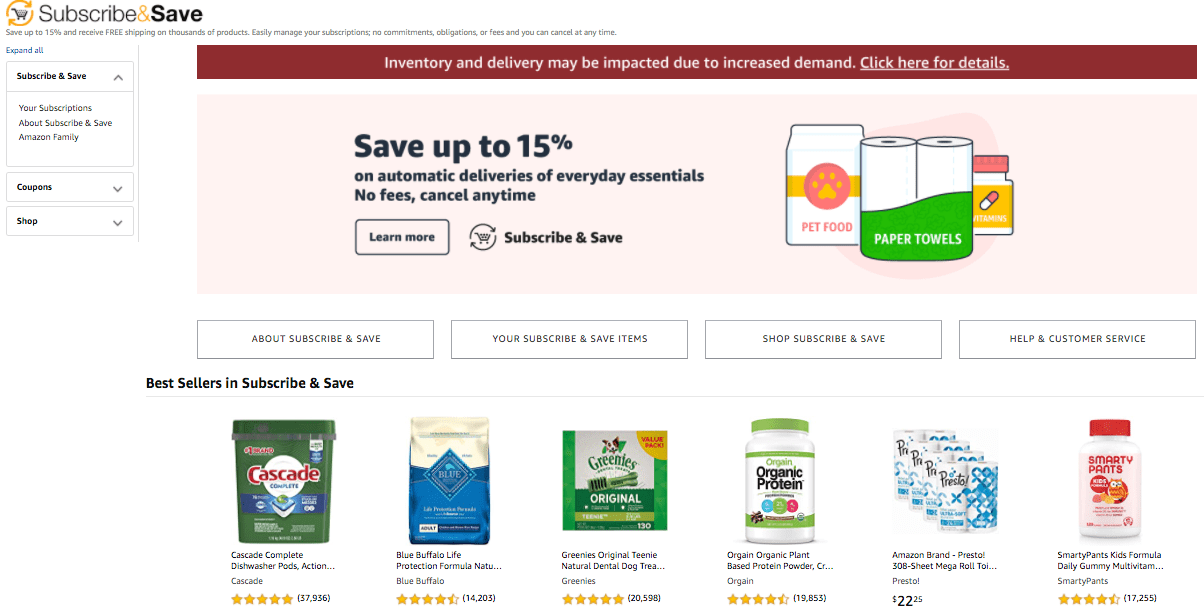This screenshot captures the "Subscribe & Save" page on Amazon. In the upper left corner, prominently displayed in bold text, is the phrase "Subscribe & Save." Directly beneath this, a description reads: "Save up to 15% and receive free shipping on thousands of products. Easily manage your subscriptions. No commitments, obligations, or fees. You can cancel at any time." The page further elaborates on "Subscribe & Save," featuring user options for managing subscriptions, learning about the program, exploring Amazon Family benefits, and accessing coupons and shopping links.

A red banner spans across the page, warning users: "Inventory and delivery may be impacted due to increased demand. Click here for details." Positioned on the right side is an image showcasing a bag of pet food, two rolls of paper towels, and a bottle of aspirin, accompanied by the text: "Save up to 15% on automatic deliveries of everyday essentials. No fees, cancel anytime." A button labeled "Learn More" is prominently placed below this statement.

Just underneath, the "Best Sellers in Subscribe & Save" section is presented, featuring images of six popular products in a horizontal row. The first product is Cascade dishwasher pods, accompanied by its average star rating and the number of reviews. Next to it is an image of Blue Buffalo pet food, followed by Greenies dental dog treats. The fourth product depicted is Orgain organic plant-based protein powder. The fifth item is Amazon brand Presto bath tissue, and the final product is SmartyPants kids multivitamins.